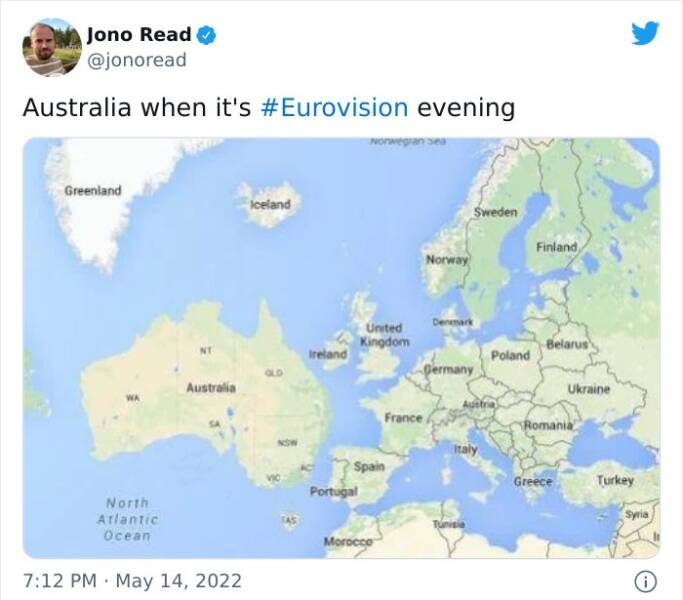The image is a screenshot of a tweet by Jono Reid, a verified user with a blue checkmark next to his name and the handle @JonoReid. His profile picture appears at the top left, showing a white male with a goatee, wearing a green and white striped shirt, with a backdrop of trees and grass. The tweet, dated May 14, 2022, at 7:12 PM, humorously states, "Australia won its #Eurovision evening." Alongside the tweet is a map of Europe that humorously places Australia in the North Atlantic Ocean, right next to Ireland, the UK, France, and Portugal. The map features typical colors for land and water, with Australia oddly superimposed next to the European countries. The Twitter bird icon is in the top right of the screen, and a small informational icon, resembling an eye inside a circle, is at the bottom right.